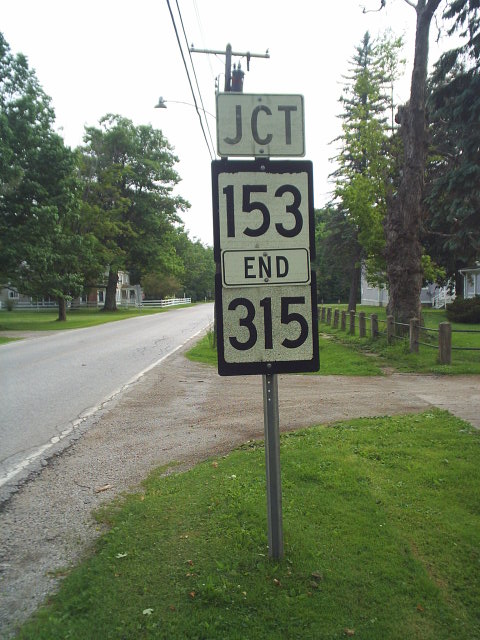The image captures an overcast outdoor scene showcasing a junction road sign against a white sky backdrop. In the middle of the photograph, a silver-colored metal pole supports two road signs. The top sign has "JCT" printed in gray letters on a white background. Below it, a second sign displays the numbers "153" and "315" along with the letter "N" in black text. The road sign stands on a green grassy patch adjacent to a paved road. Trees line the road, with electrical wires and a streetlamp visible overhead. On the right side, a wooden fence is present, and there are medium-sized, white-painted wooden homes flanking both sides of the road.